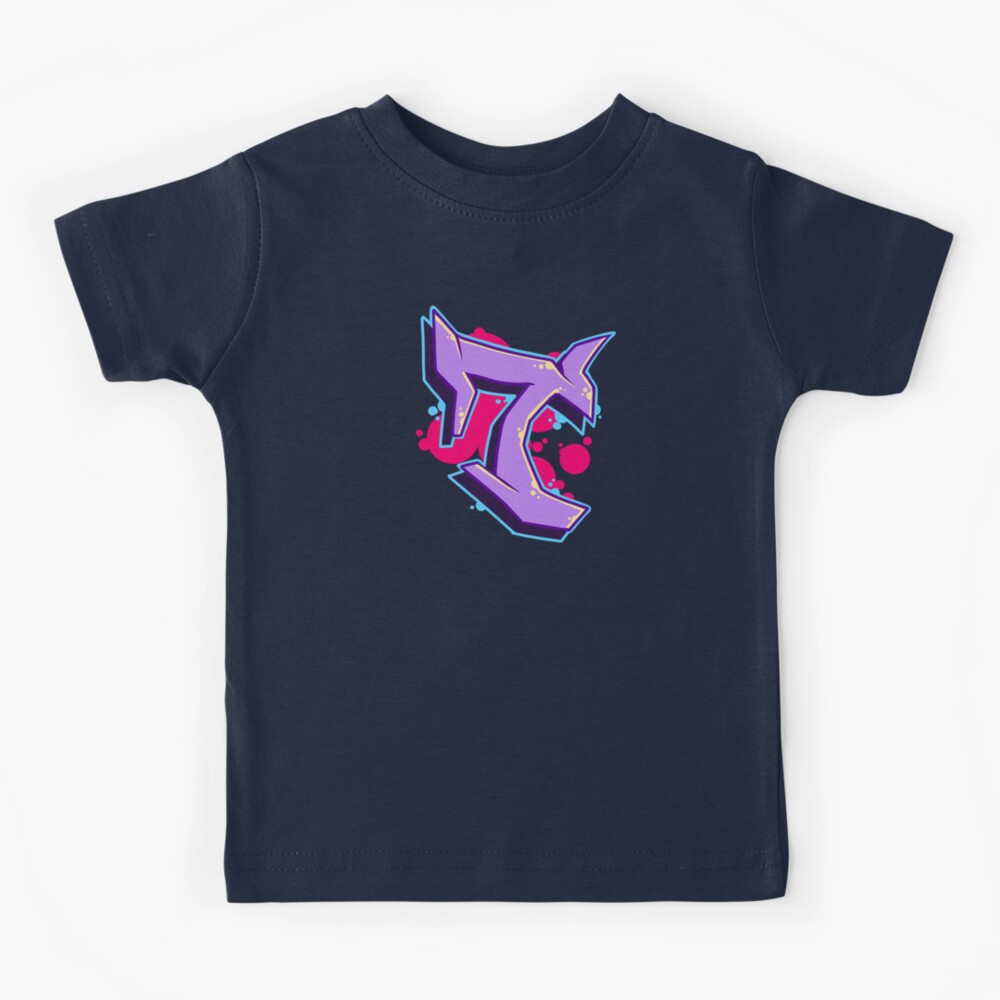This black t-shirt features a striking graffiti-style design prominently displayed in the center. Dominating the shirt is a prominent numeral "7" rendered in a light purple 3D font, giving it a glossy and textured appearance. Enhancing its visual impact, the "7" is intricately outlined with a light neon blue border. Behind the numeral, a dynamic splash of hot pink, along with additional splashes of blue, adds depth and vibrancy to the graphic. The overall design embodies a bold and edgy graffiti aesthetic against the stark contrast of the black fabric. The shirt is showcased on a plain white background, highlighting its unique and contemporary urban art style.